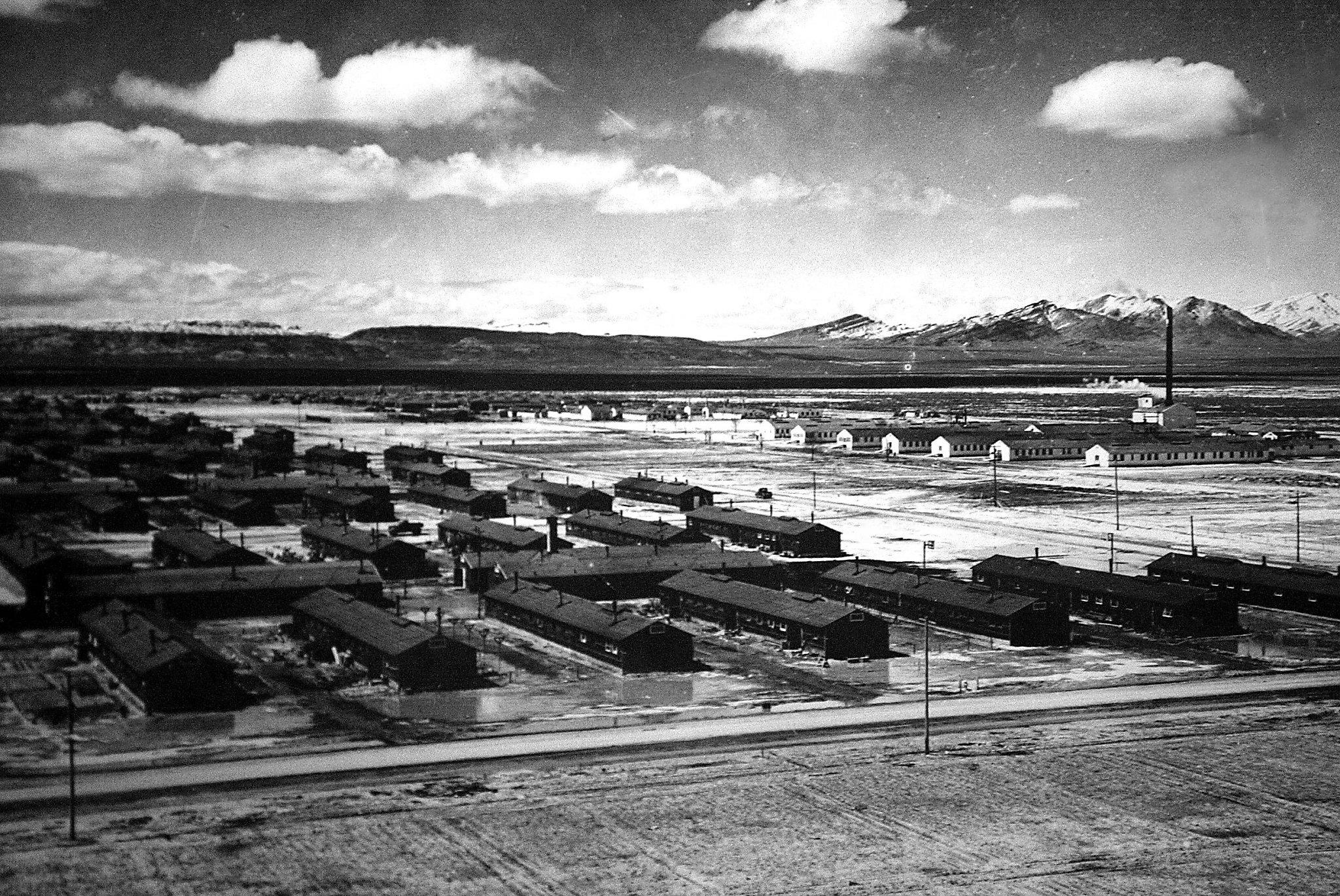This black-and-white photograph depicts a vast, remote landscape possibly suggesting a military base, internment camp, or old campsite. The terrain is flat and appears flooded, with puddles scattered across the ground. The image captures an array of long, single-story buildings aligned in rows, characterized by their dark color and windows running down their sides. These structures have roofs that slant downward from a straight ridge at the top. In the distance, snow-capped mountains rise, particularly prominent on the right. Towards the right side, there’s a distinctive building with a tall chimney or smoke stack. The photograph, devoid of any additional context, highlights the isolation and extensive sprawl of the complex against the vast and open terrain.